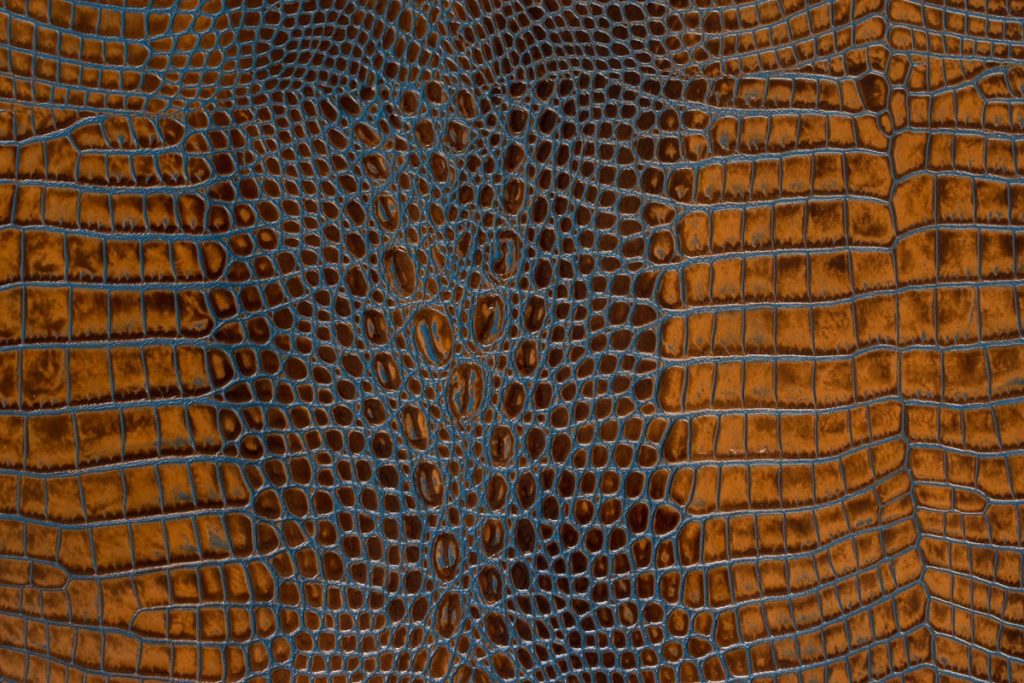The image depicts a close-up view of a textured surface that seems to be alligator hide or a similar type of leather. The background is predominantly bronze or orange-brown, accentuated with darker spots, giving it a rich, varied hue. Prominent are gray, thread-like veins crisscrossing the surface, creating a netted pattern that overlays the bronze backdrop. This netting effect makes it look as though there are rectangular and circular patterns scattered across the surface, with the rectangles morphing into circles near the center of the image. The image is horizontally framed and rectangular, capturing the intricate details of what appears to be skin or material, possibly leather, with a textured, scale-like appearance akin to lizard or alligator hide.